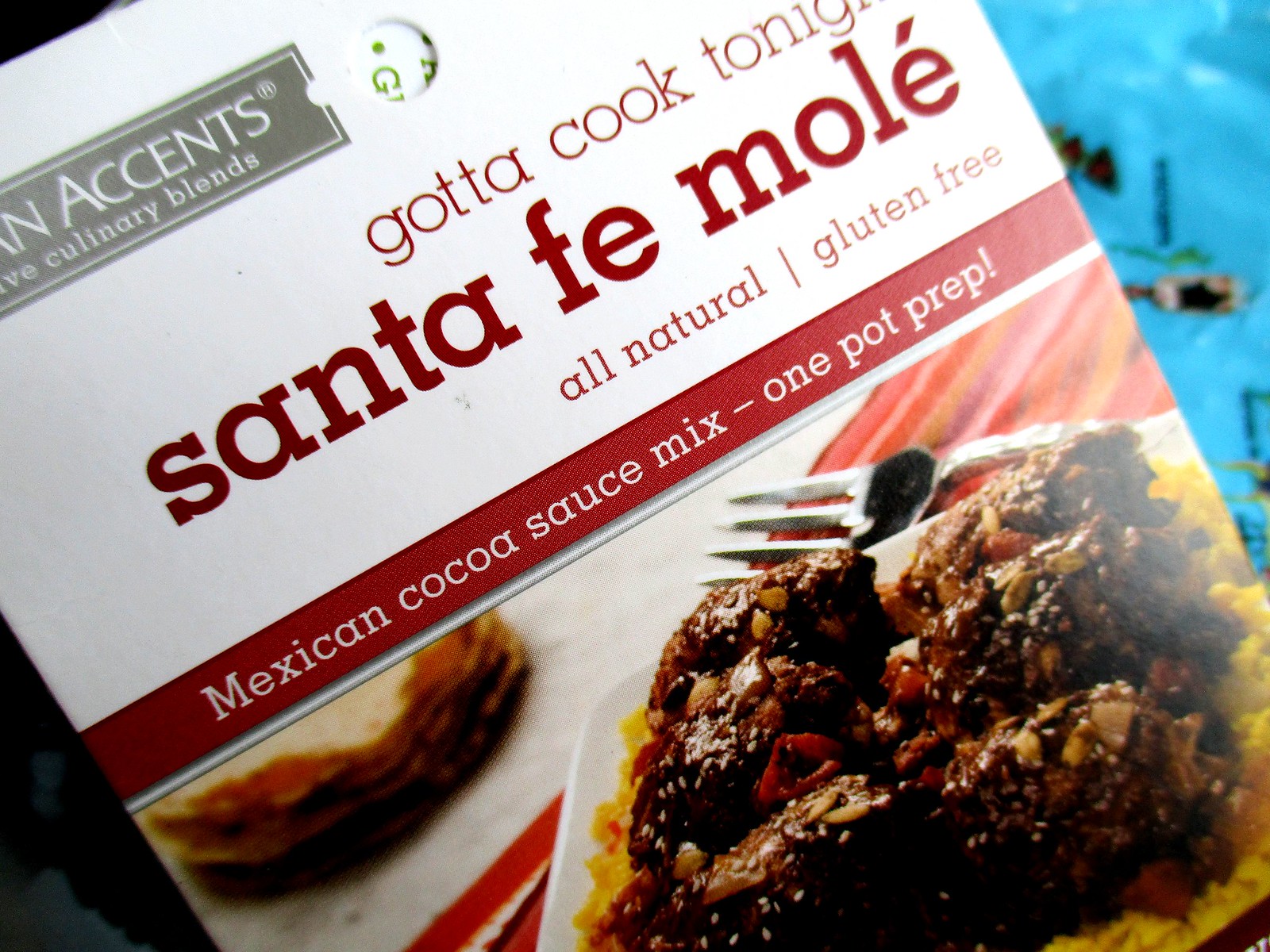The image is a close-up of a food product packaging, predominantly white with a small gray bar at the top that reads "accents" and possibly "culinary blends." Below, in red text, the slogan "Gotta cook tonight?" is prominently displayed, followed by the product name "Santa Fe Molé." Further down, it highlights attributes such as "All natural" and "Gluten-free" in separate sections. A prominent red bar spans across the middle, declaring in white text, "Mexican Cocoa Sauce Mix - One Pot Prep!" Beneath this, an appetizing image showcases the product—a brown dish garnished with a variety of peppers and onions, placed adjacent to a silver fork. The fork appears to rest on a red and white tablecloth adding a touch of color and context to the culinary presentation.